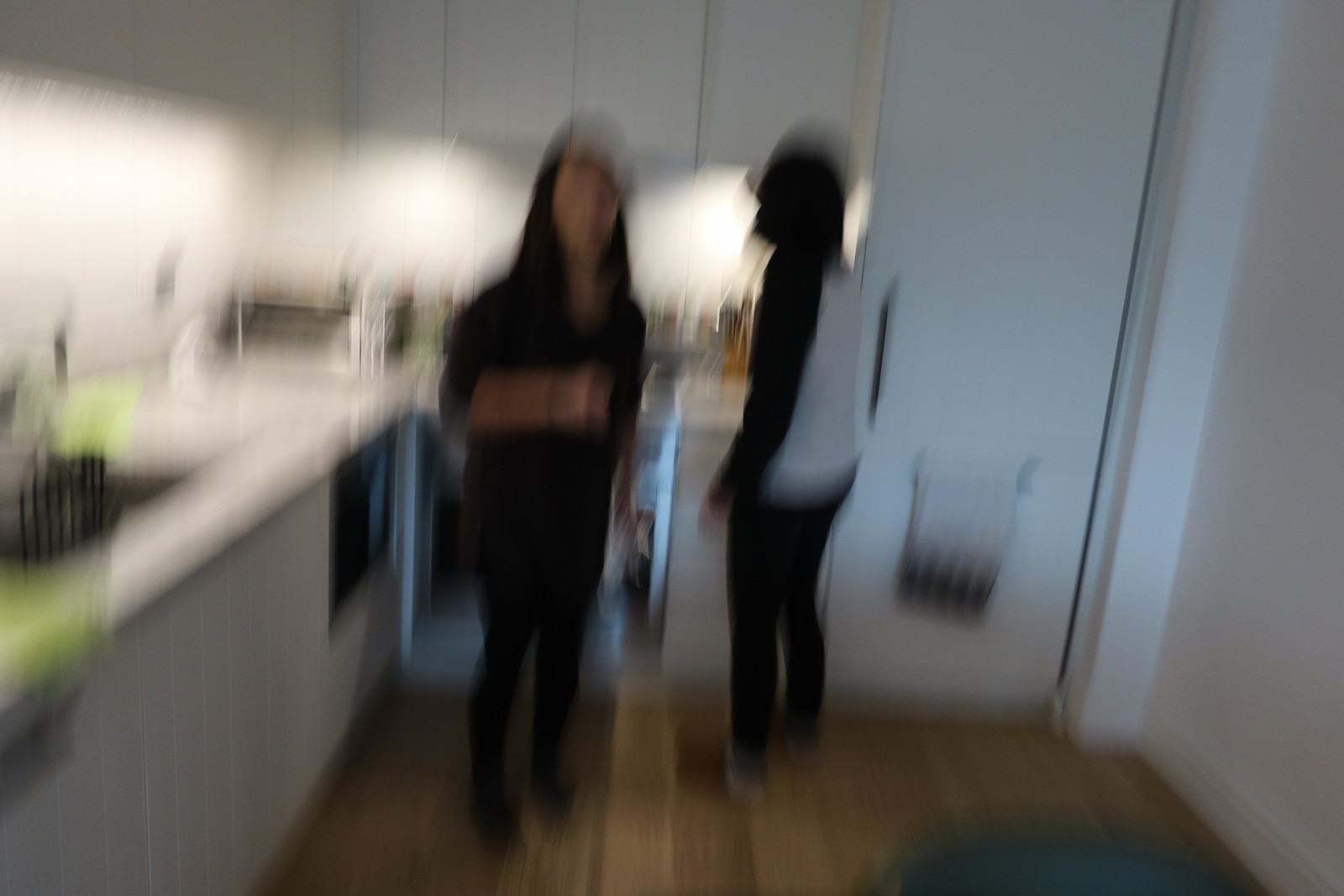In this extremely blurry photograph of a kitchen, two indistinguishable individuals are depicted. The kitchen features a brown wood floor and a blue rug, with white kitchen counters, cabinets, and backsplash. A silver stove and oven combination is visible, and to the left, a long counter with a sink and lime green accents, whose details are unclear, stands out. The back counter is adorned with a toaster oven and various cooking supplies. The person on the left, dressed entirely in black with dark hair, faces the camera, while the person on the right, clad in black pants and a white and black shirt, has shorter dark hair and faces away.